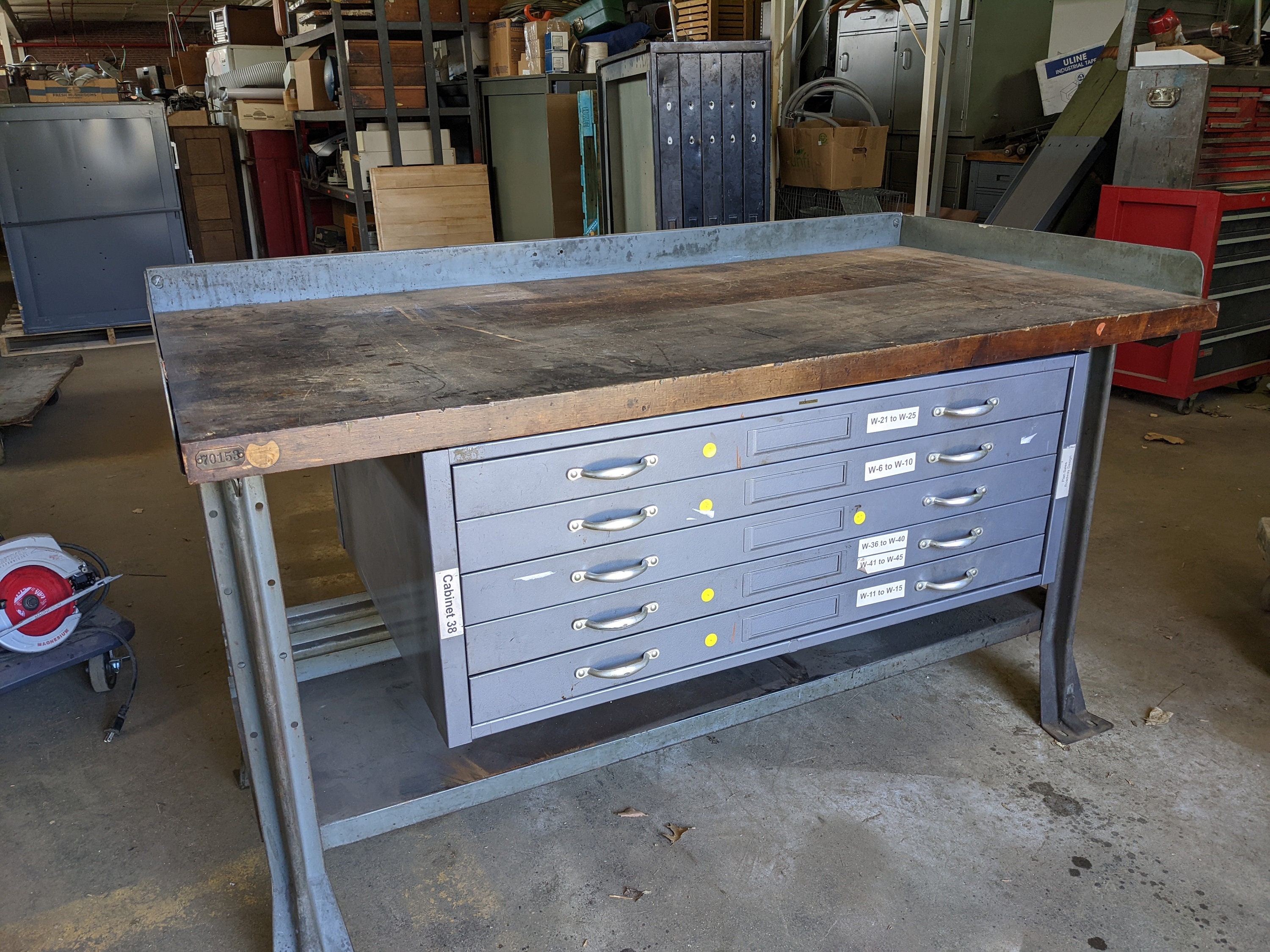The image depicts the inside of a garage workshop, centering around a large, robust workbench. The workbench has a thick wooden top with a steel railing around the edge, designed to prevent items from falling off. Below the wooden top, there is an organized array of metal drawers—two columns with five rows each. The drawers are a gray color, equipped with silver handles, and some on the right are labeled. The entire structure is supported by steel legs, and there's an additional steel shelf at the bottom for extra storage. To the left of the workbench stands a skill saw mounted on a wheeled cart, while the background reveals more shelves and cupboards, cluttered with various items such as cardboard boxes and possibly even doors. The tarnished, well-used appearance of the workbench and contents suggests a highly active and functional handyman's shop.